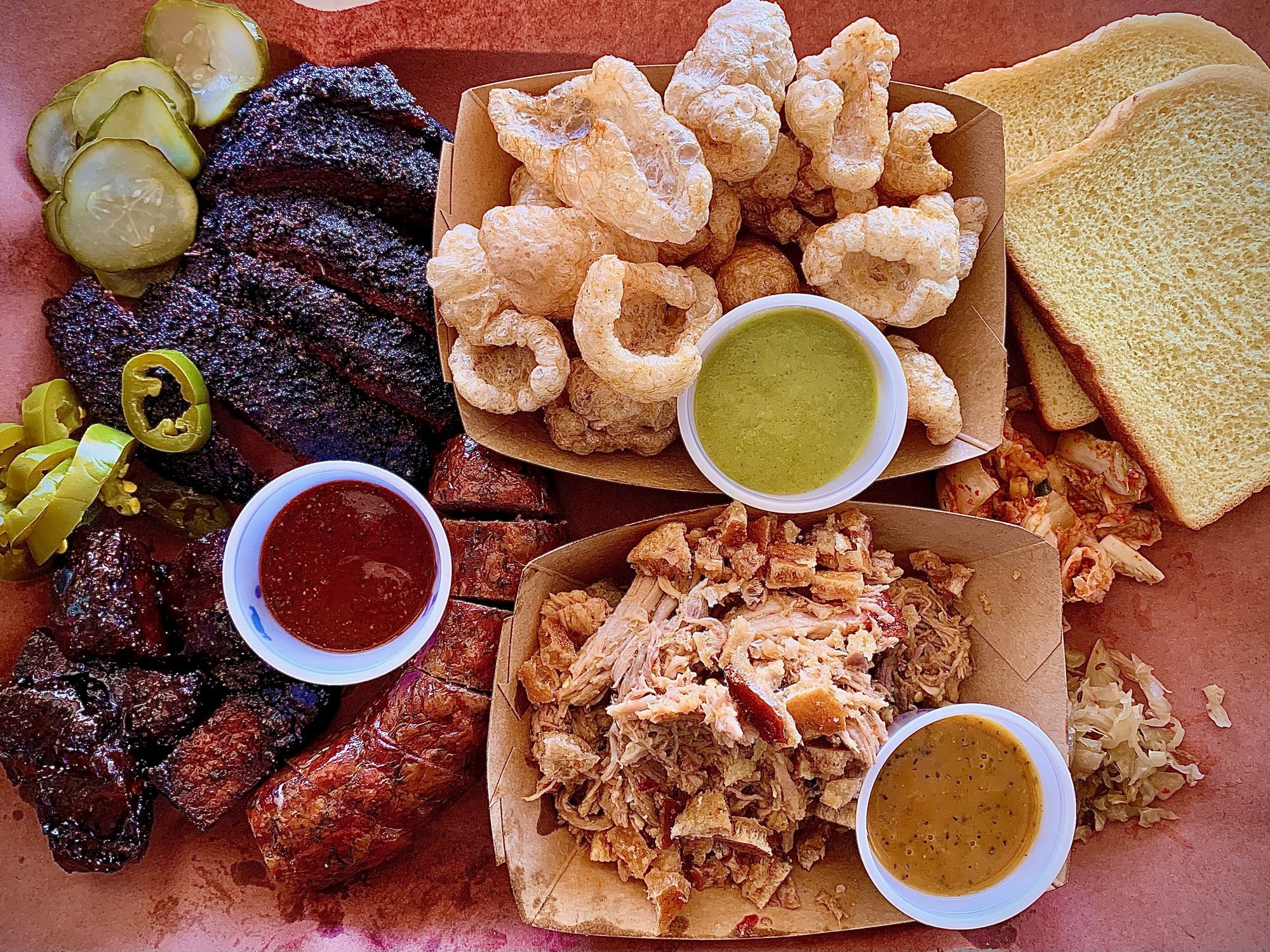This overhead photograph captures a richly detailed spread of food on a table with a burnt orange hue. Central to the image are various items typical of a hearty barbecue meal. On the left, there's charred brisket, pink on the inside, accompanied by sliced jalapeños and cut-up pickles. Nearby, white bowls contain three types of sauces: a red ketchup, an orange habanero sauce, and a green salsa. Right of this section, there's a portion of sliced sausage beside a cardboard container holding shredded chicken. Above the chicken, a pile of crispy pork rinds is placed. Adjacent to the pork rinds, another white bowl features a yellow sauce. To the rightmost position, there are two slices of light brown bread with a side of fried onions below them. The food items, showcasing colors from blackened meats to vibrant green pickles and an array of sauces, are positioned in separate containers, each meticulously arranged to present a visually appealing and mouth-watering scene.